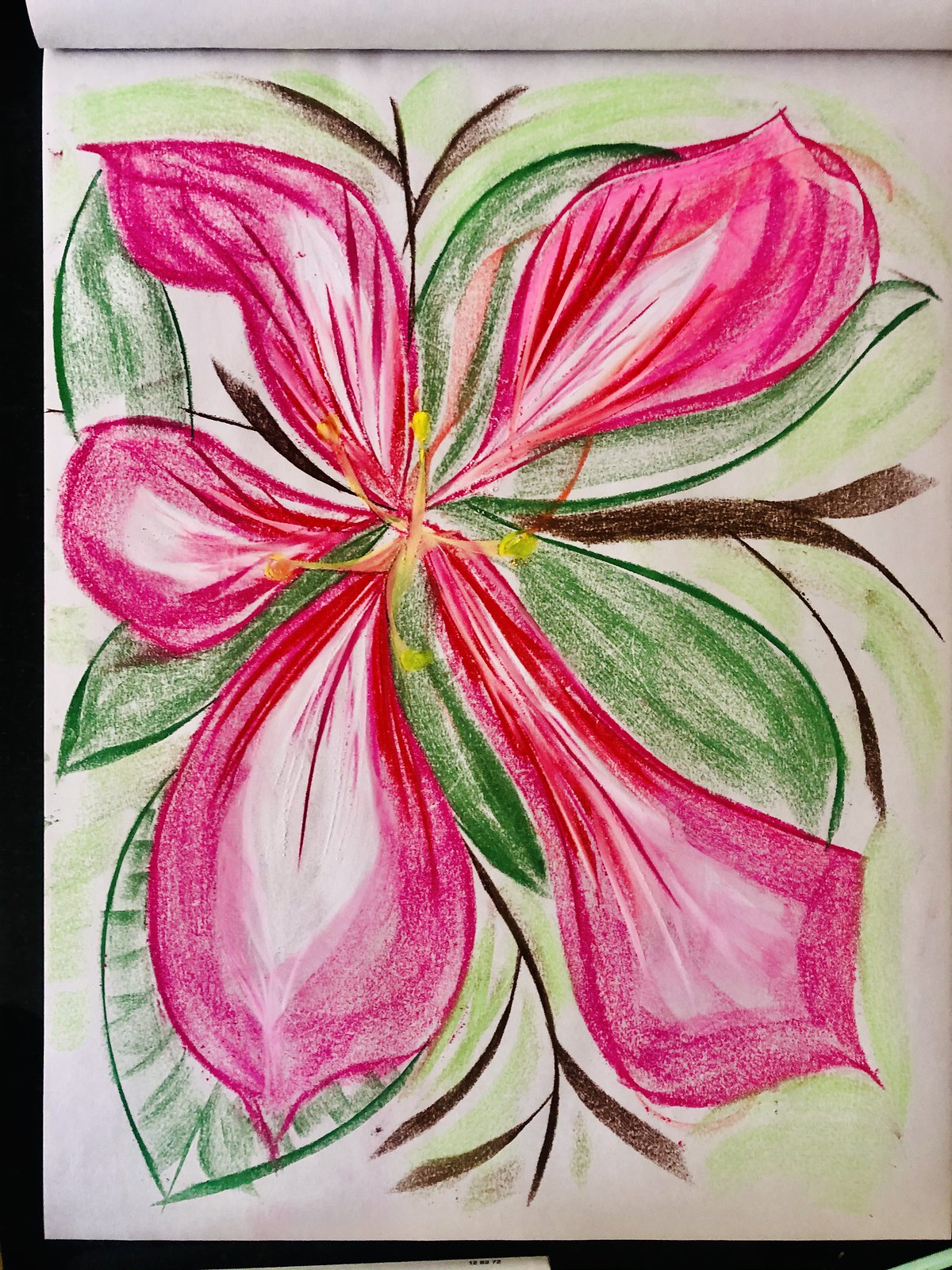This image features an artistic drawing on folded drawing paper, showcasing a large, detailed flower that almost fills the entire canvas. The flower, predominantly colored in shades of pink and green, exhibits vibrant yellow in its central part. Surrounding the bloom are green leaves, enhancing its natural beauty, and brownish branches extend from the top and right sides of the flower. The drawing's backdrop includes a dark area on the left and the bottom, hinting at the paper's resting surface. The image is devoid of any text or additional elements, focusing solely on the remarkable floral illustration.